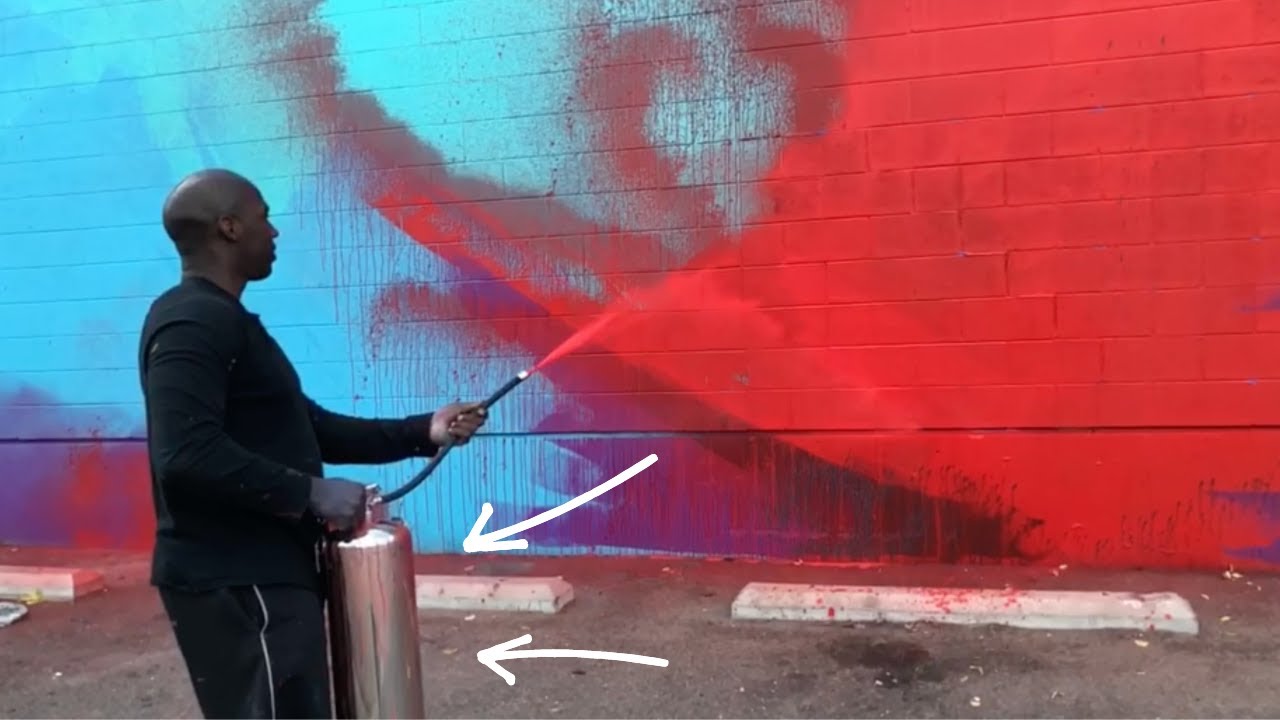This photograph captures a scene where a man with dark skin, dressed in a black jacket and black pants, is engaged in spraying red paint onto an exterior wall of a building. He holds a silver canister in his right hand, with a thin black hose extending from it, which he grasps with his left hand. The hose emits a mist of red paint that blends into the brilliant blue and purple hues already present on the wall. The entire setup, including the manually superimposed white arrows pointing to the silver canister, suggests a focus on the equipment he is using. The wall, part of a building located in a parking lot, showcases a vivid transformation as the red paint intermingles with the original colors, hinting at artistic intentions. The scene is vibrant with the contrast of the shiny silver tank, the striking red spray, and the colorful wall backdrop, illustrating the process of what appears to be the creation of a large, vivid mural.